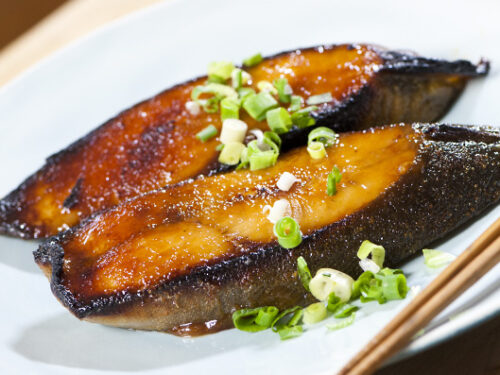A closeup image features a white plate with two pieces of what appears to be Japanese cuisine, possibly eel sashimi. Each piece is approximately three inches long and has a sliced top with an orangish-yellow hue, transitioning to a brownish, blackish, or grayish skin on the sides. Chopped green onions are artfully sprinkled over the sashimi and a portion of the plate. In the top right corner, plain wooden chopsticks are positioned diagonally, adding to the culinary presentation. The overall composition highlights the intricate details and textures of the dish.